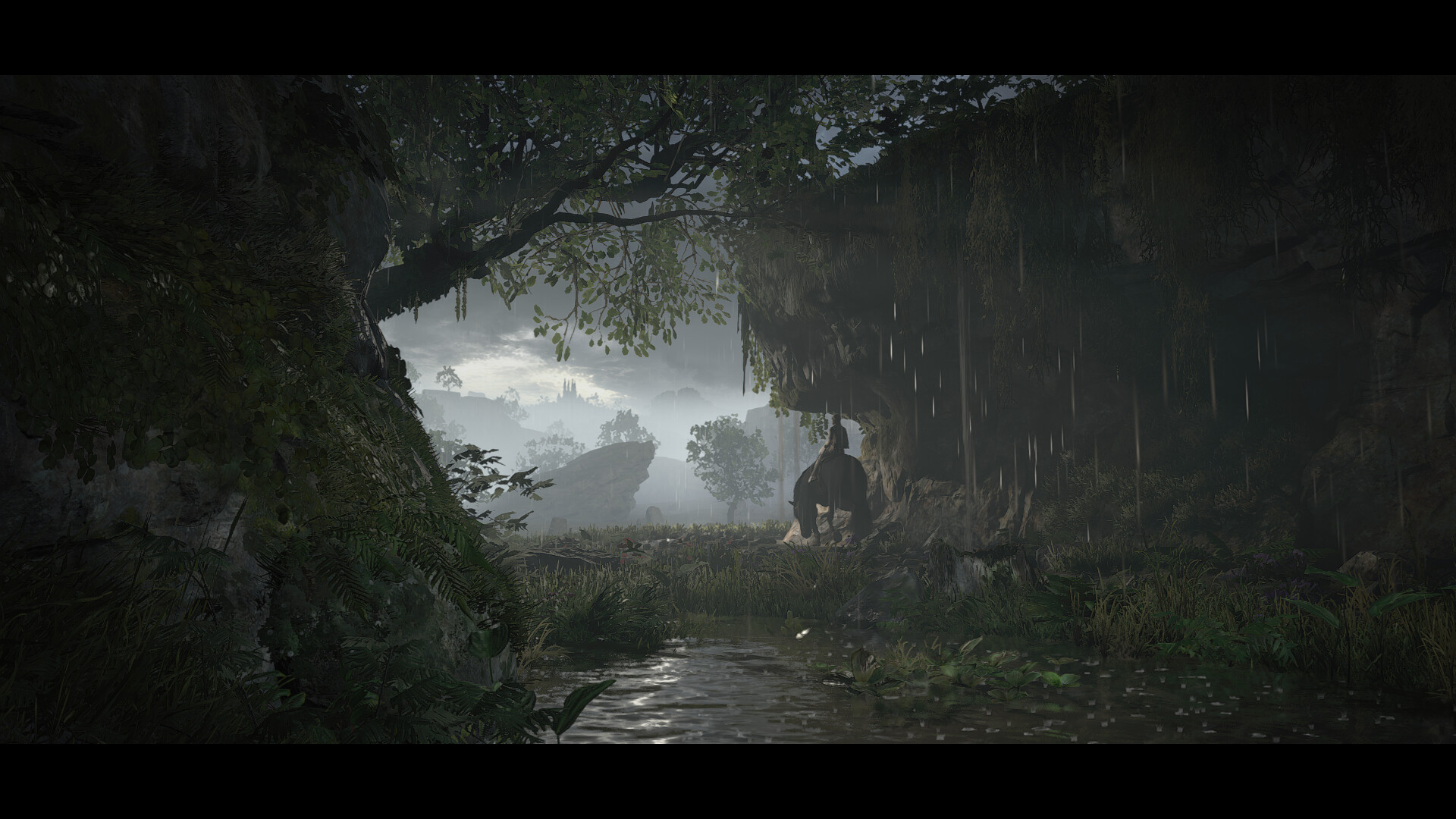A somber, dystopian scene from a video game portrays a dark and dreary atmosphere. At the center of the image, a solitary figure sits atop a horse, both appearing weary with the horse's head hanging low. Rain drips steadily, cascading down into what seems to be the entrance of a cave. The background is enveloped in a thick mist, subtly revealing a grand, rocky outcrop reminiscent of the iconic scene from The Lion King. Far in the distance, a faint silhouette of a castle emerges through the haze, adding an element of intrigue and desolation to the landscape.